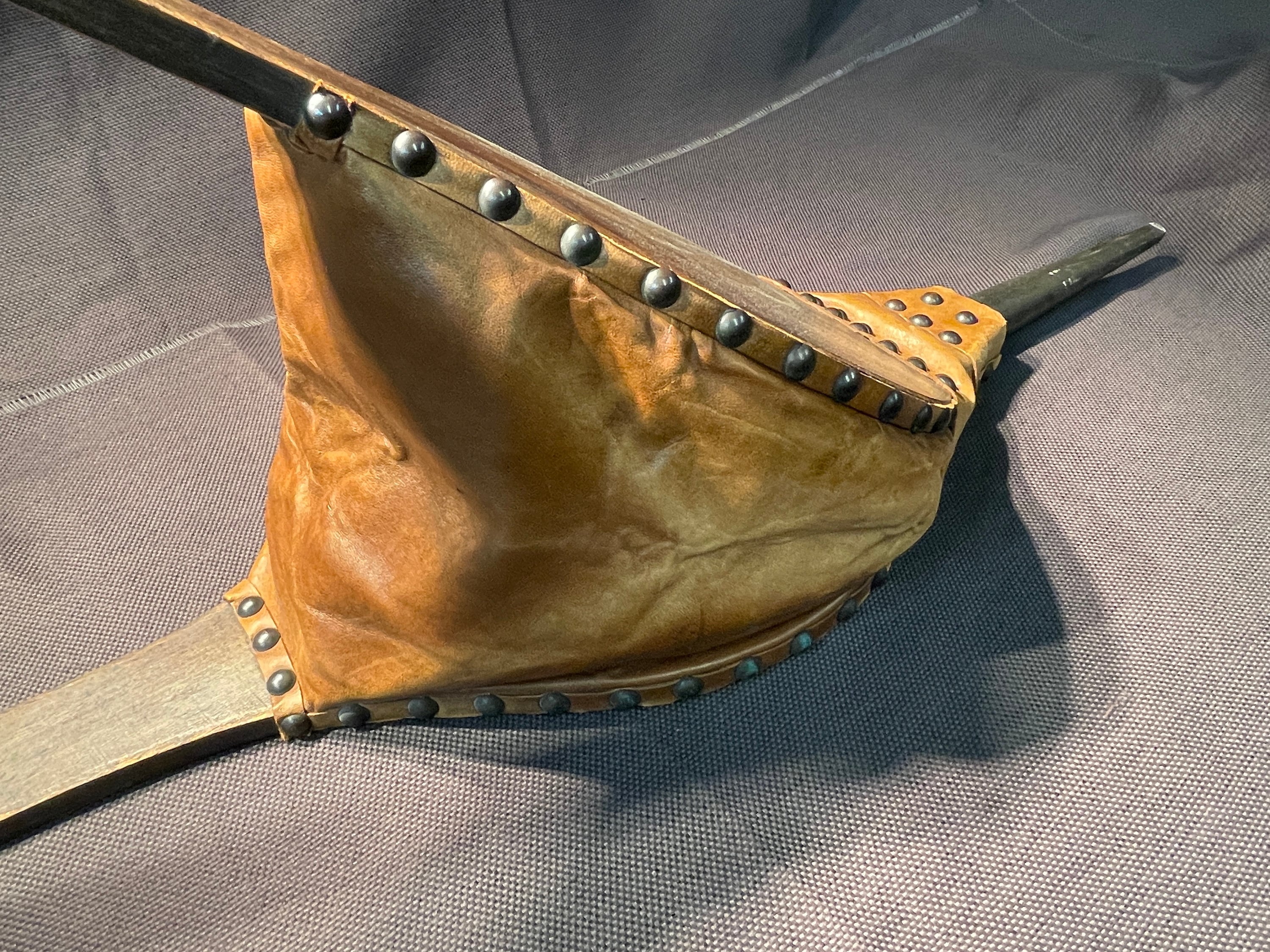This detailed photograph showcases an antique fireplace bellow, likely used for a forge or fireplace, displayed on a grey canvas surface. The bellow features two wooden paddles with clean, dark wood handles that fan out and are connected at the ends by a smaller piece of wood. Brass studs line the edges of the bellow, adding a touch of craftsmanship. A black rod protrudes from the connecting piece. The bellow itself is crafted from soft, suede-like brown leather, displaying a mix of dark and light brown hues. Despite its antique design, the leather appears fresh and well-maintained, indicating its readiness for use or simply as a pristine collectible. The overall scene suggests that the item is being exhibited for sale or display.